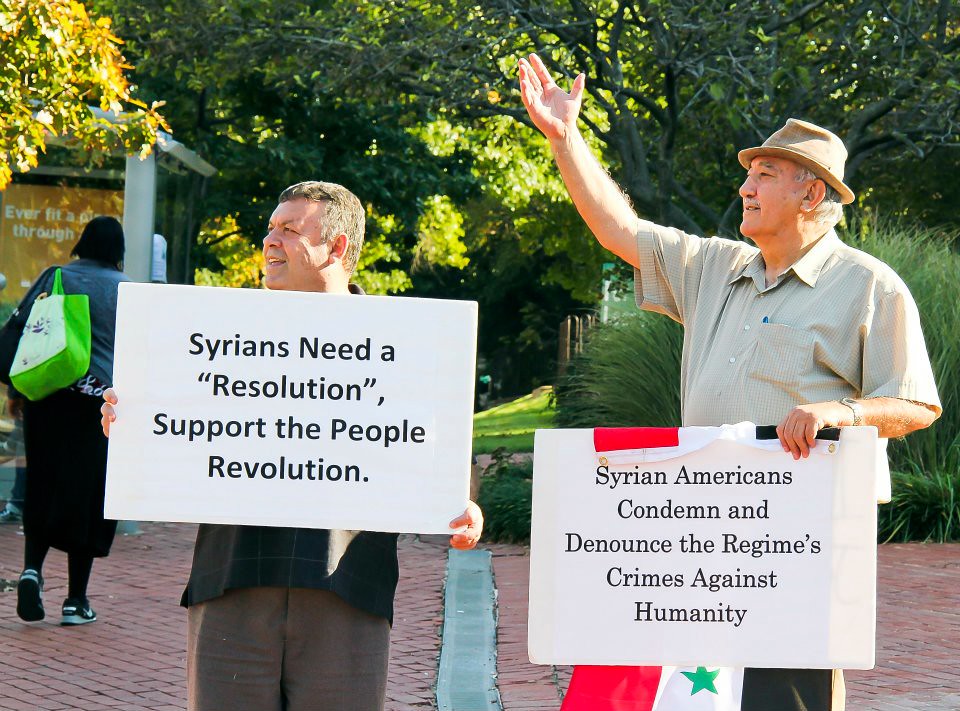In a vibrant outdoor setting adorned with lush, varied green trees and plants, two men are passionately protesting on a street corner. The backdrop features a picturesque mix of dark and light green foliage, with a thick bush exhibiting long green leaves to the right. On the left side, near the edge of a bus station with a visible billboard, a woman with a backpack walks away from the camera, adding to the bustling atmosphere.

The man on the left is relatively short and dressed in a black shirt with brown pants. He holds a large white rectangular sign that reads, "Syrians Need a Resolution, Support the People Revolution" in bold black font. His companion on the right wears a brown polo shirt and a brown hat, gesturing emphatically toward the top left corner. He holds a white piece of paper inscribed with "Syrian Americans Condemn and Denounce the Regime's Crimes Against Humanity."

Both men exhibit a strong sense of purpose, with the man on the right raising his arm, possibly to attract attention from passersby or vehicles. A flag with red, black, and white stripes and green stars is partially visible behind his sign, further emphasizing their cause. The scene, bathed in bright sunlight, hints at a lively, park-like ambiance, though the exact size of the crowd remains unclear. Nonetheless, these two determined protesters stand out prominently, advocating for the end of the Syrian regime's atrocities.